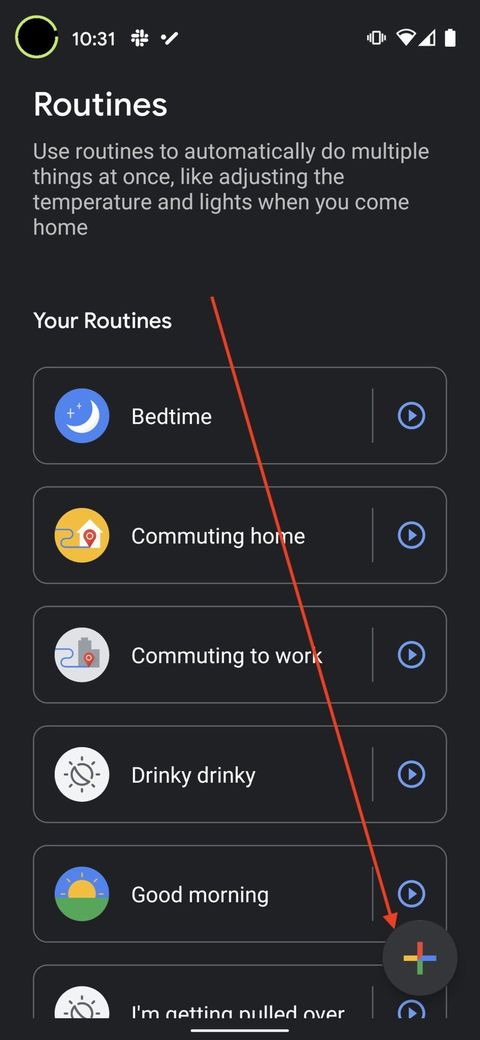A detailed screen capture from an iPhone displaying an automation app in focus. At the top, the standard iOS status bar is visible, which shows the signal strength, battery level, and the time. Central to the screen, the app's interface is laid out, beginning with a white-font header in the upper left corner that reads "Routines." Below the header, there's an informative blurb explaining the app's functionality: "Use routines to automatically do multiple things at once like adjusting the temperature and lights when you come home."

Further down, the section titled "Your Routines" introduces a list of pre-configured routines, each housed in distinct rectangular blocks. The routines listed are:
1. "Bedtime"
2. "Commuting Home"
3. "Commuting to Work"
4. "Drinky Drinky"
5. "Good Morning"

Superimposed on the app interface is an overlay featuring a thin red line with an arrowhead, extending diagonally from the upper center towards the lower right corner. This red line points to a small black circle containing a multicolored cross. This circle likely represents the button where users can edit or add new routines.

To the right of each routine block, there appears to be an edit button, suggesting that users can customize the predefined routines to better suit their needs. This screen capture provides a clear and comprehensive visual of the app's capacity to manage and automate daily tasks conveniently through a smartphone.